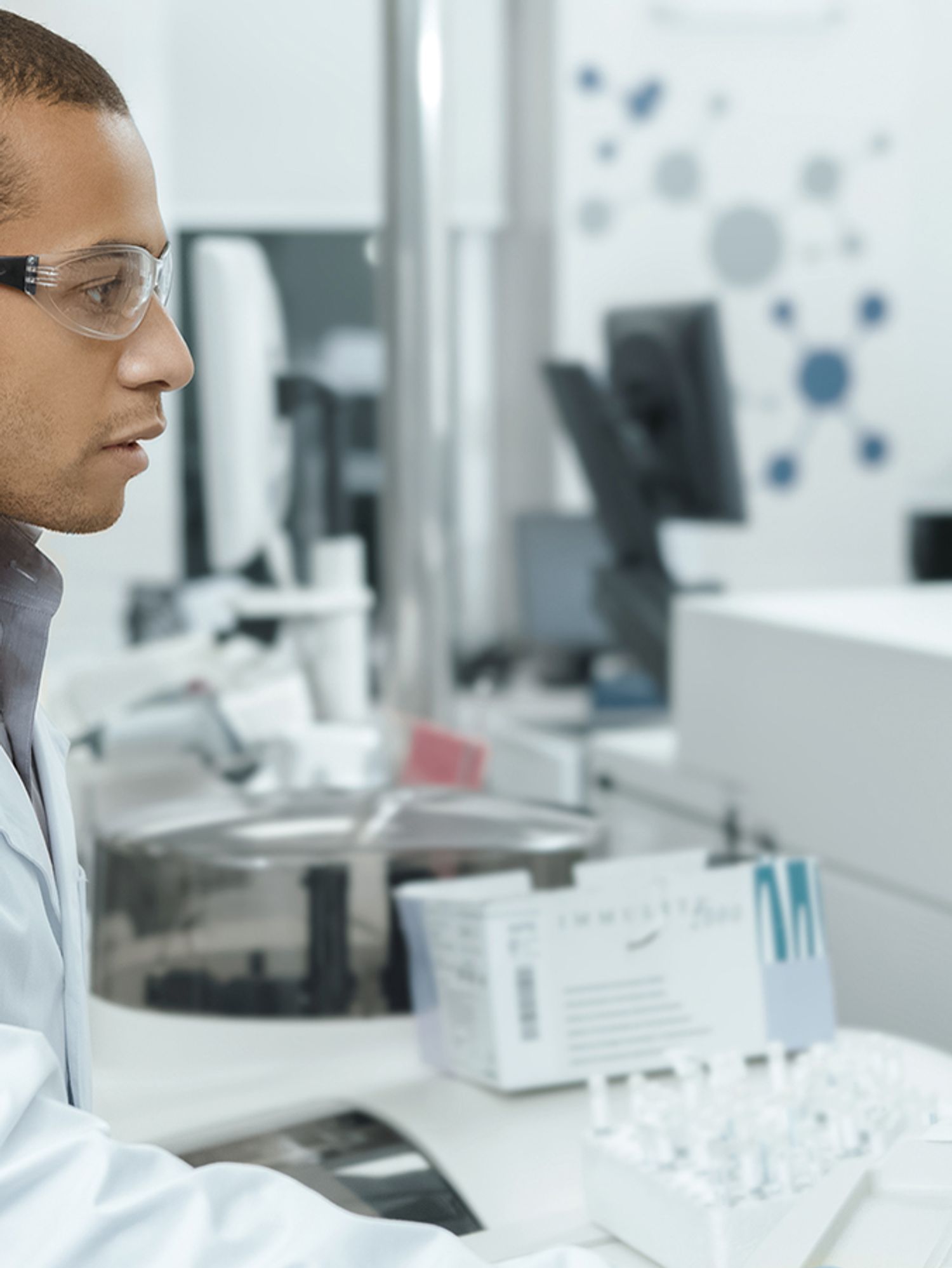The color photograph depicts a young African American scientist in a laboratory, partially cut off by the left edge of the image in a portrait orientation. The man's right side of the face is clearly visible, and he appears to be in his 20s, focused on something out of the frame. He wears safety goggles and a white lab coat, suggesting a professional and safe working environment. His right arm extends onto the lab workstation, which holds a variety of scientific apparatus, including a test tube drying rack and a tray for samples. 

A partially obscured piece of lab equipment with a smoke-gray plastic lid, possibly a sample spinning device, is also present on the bench. In the blurred background, there are two computer monitors and various laboratory gear, including stainless steel and white metal equipment. The lab's back wall is adorned with stickers resembling molecular diagrams, adding a touch of scientific decoration. The predominant color in the photograph is white, highlighting the sterile and orderly environment typical of a scientific or medical lab.